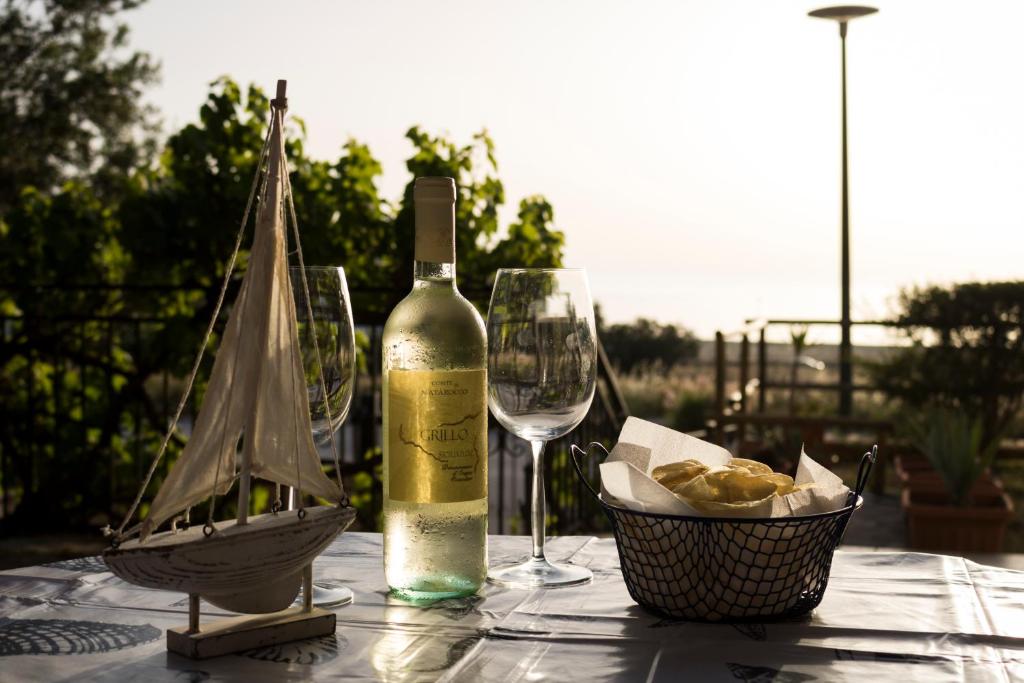The image captures an elegant outdoor setting, possibly a vineyard or a deluxe garden, where a wine bottle and two empty wine glasses are prominently displayed on a table covered with a vinyl tablecloth. The table also features a decorative model sailboat, adding a whimsical touch. Accompanying the wine are tortilla chips or bread in a black, see-through bowl. The background is lush with greenery, including numerous trees, garden beds, planters, and supports likely for grapevines. An outdoor heater or light fixture resembling a streetlight stands in the backdrop. The scene, with its detailed elements and rich ambiance, evokes the feel of a romantic date night or a serene restaurant patio, with the focus squarely on the table's contents.